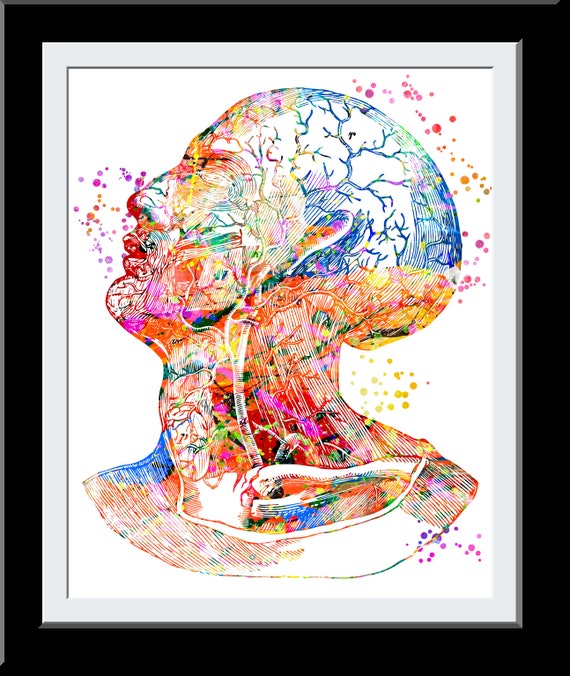The image features a detailed art print with a sophisticated framing. The outermost border is black, followed by a grayish-white mat, leading into a white background that emphasizes the central artwork. The artwork itself is a vividly colored depiction of a human skull and upper body, focusing particularly on the head, neck, and upper chest. The human figure is shown in profile, gazing slightly upwards and with the mouth slightly open. The skin is rendered transparent, revealing intricate anatomical details such as veins, neck muscles, and the ribcage. The brain appears predominantly blue with a mix of greens, reds, and purples, while the face and neck display a spectrum of reds, blues, greens, purples, and yellows. This colorful composition extends to the surrounding space, with splotches and dots of various colors—blues, purples, yellows—scattered around the mouth, base of the head, and the top of the head. The image artistically captures the complexity of human anatomy and the vibrancy of neurological and vascular processes.